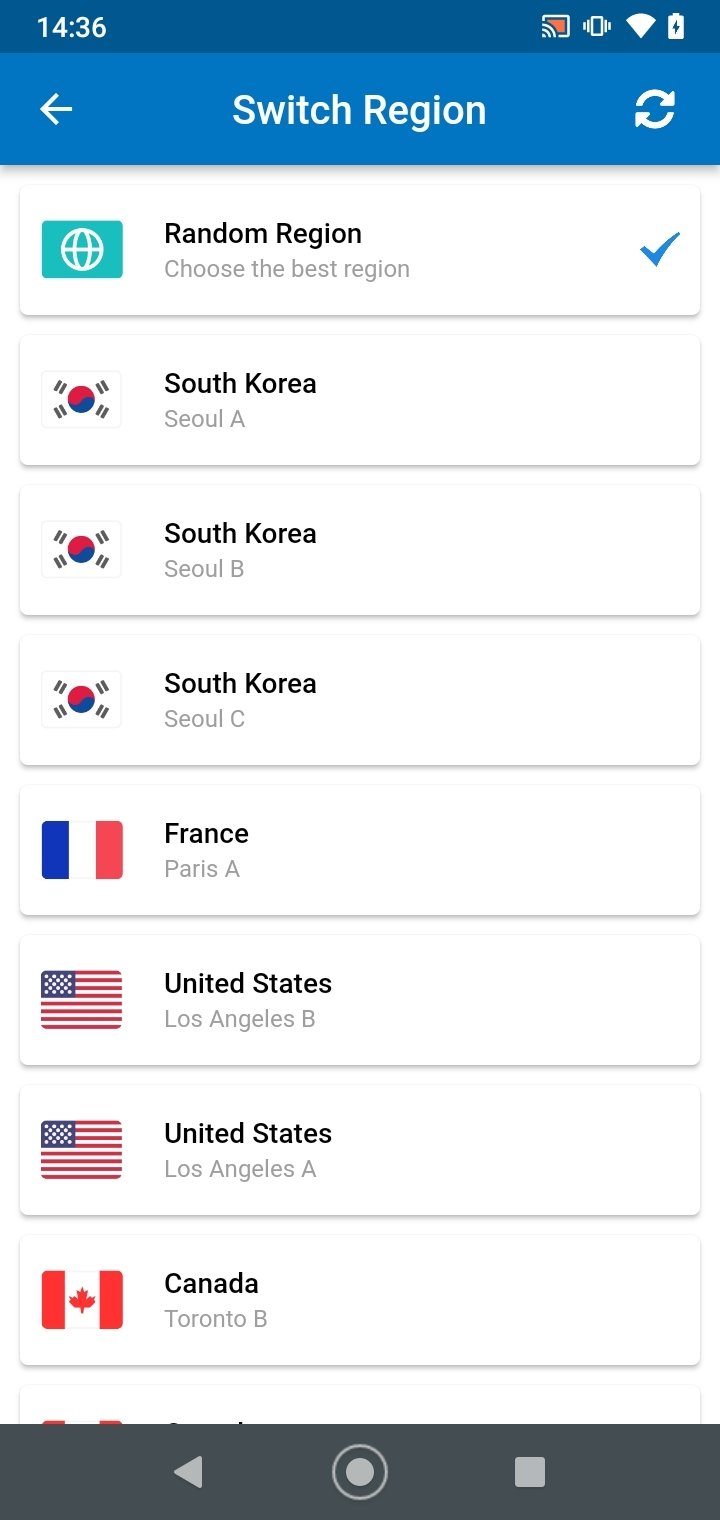The image appears to be a screenshot from a mobile device. At the very top, a blue status bar displays "1436" in the upper left corner, with icons on the right indicating Wi-Fi, battery level, and vibration mode. Below the status bar is a lighter blue section featuring a left-pointing arrow labeled "switch region," alongside two circular arrows forming a refresh symbol.

In the main portion of the screen, various categories are listed vertically. At the top of the list, "random region" with the option to "choose the best region" is marked with a blue checkmark. The subsequent entries represent different regions and their respective servers:

1. **South Korea:**
   - Seoul A (indicated with a red circle and corner lines)
   - Seoul B (indicated with a red circle and corner lines)
   - Seoul C (indicated with a red circle and corner lines)

2. **France:**
   - Paris A (accompanied by a tricolor flag - blue, white, and red)

3. **United States:**
   - Los Angeles B (accompanied by an American flag)
   - Los Angeles A (accompanied by an American flag)

4. **Canada:**
   - Toronto B (accompanied by a red and white flag featuring a red maple leaf in the center)